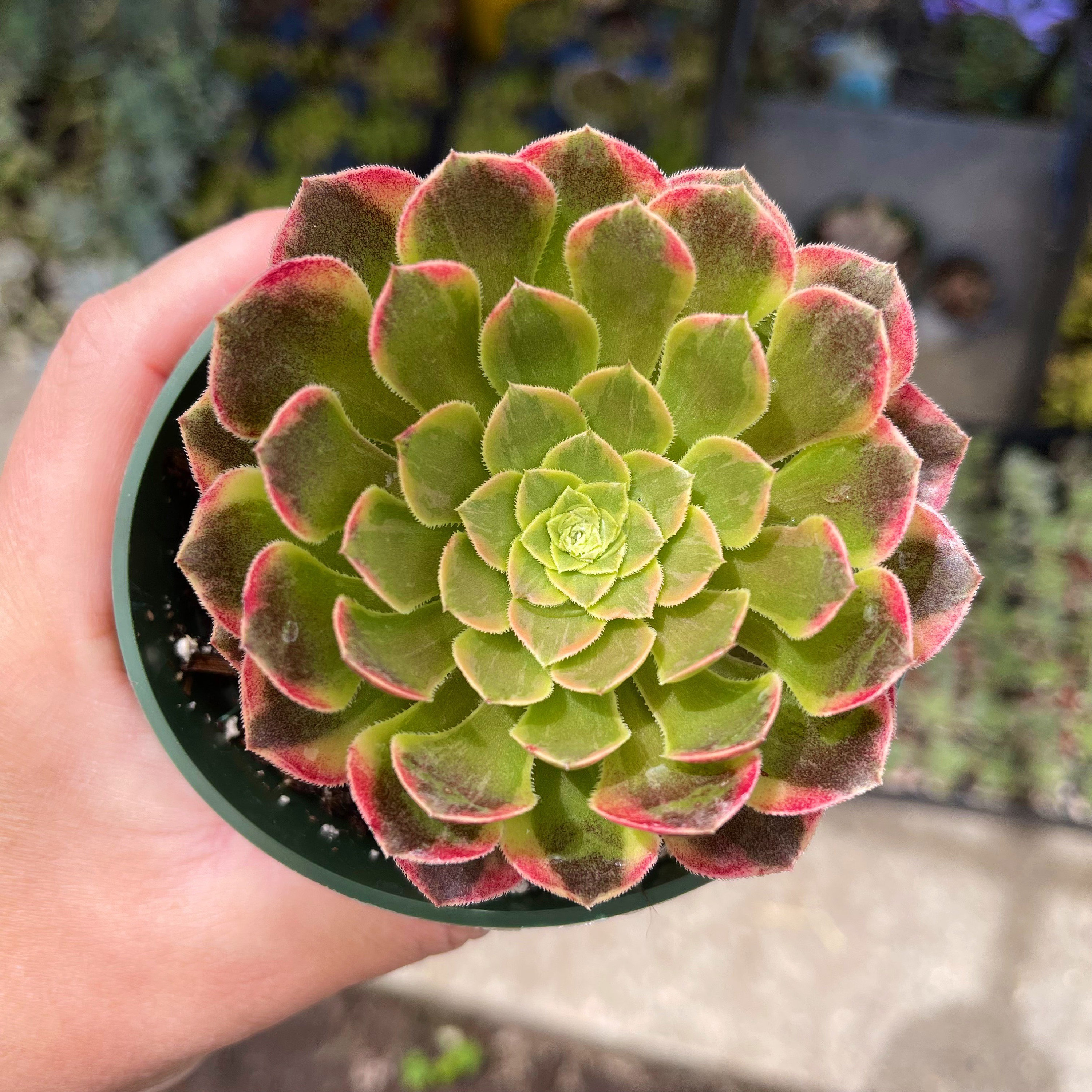This square, color snapshot captures an individual holding a decorative succulent plant, which is likely a type of cactus without thorns, in a lightly hued plastic pot. The left hand of the person is visible, securely holding the pot up to the camera. The background is indistinct, suggesting the setting could be a plant nursery or a greenhouse, hinting at a place where plants are nurtured or sold.

The succulent, akin to a lotus blossom or a rose, displays a meticulous arrangement of petal-like leaves. These leaves start small and delicate at the center and become progressively larger and more detailed towards the edges. The central leaves are a pure green, which transitions into light green and bright pink at the tips. Some descriptions suggest a reddish-purple or slightly brown shade may be evident at the outer fringes. This gradient of colors from the center to the edges enhances the plant's decorative appeal. Overall, the plant is compact, approximately the size of the holder's hand, and it stands out due to its vivid and varied hues.